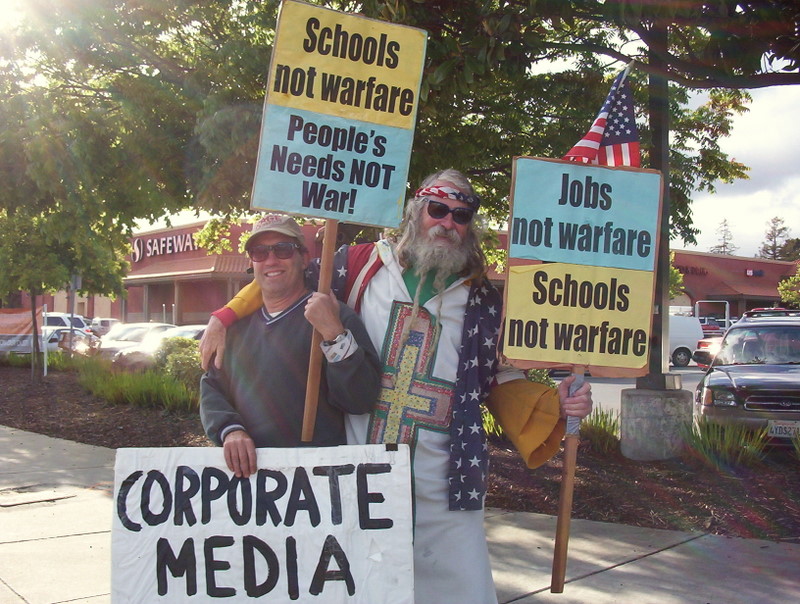In this photograph, two men are standing on a sidewalk with a parking lot and a Safeway grocery store in the background, surrounded by trees and bushes. The man on the left is wearing a tan baseball hat, a gray pullover sweater with a v-neck, dark sunglasses, and has a roll of tape dangling from his left wrist. He holds two signs: one large sign on a wooden stick that reads "Schools Not Warfare, People's Needs Not War," and a smaller sign in front of him that says "Corporate Media" in black letters. The man on the right, resembling a Vietnam veteran, sports a long white beard and long hair, and wears an American flag bandana as a headband over dark sunglasses. He is clad in a long white robe with a yellow cross on the chest and an American flag draped over his shoulders. He holds a sign that reads "Jobs Not Warfare, Schools Not Warfare." An American flag is also visible above their signs, adding to the visual impact of their peaceful protest on this street corner.